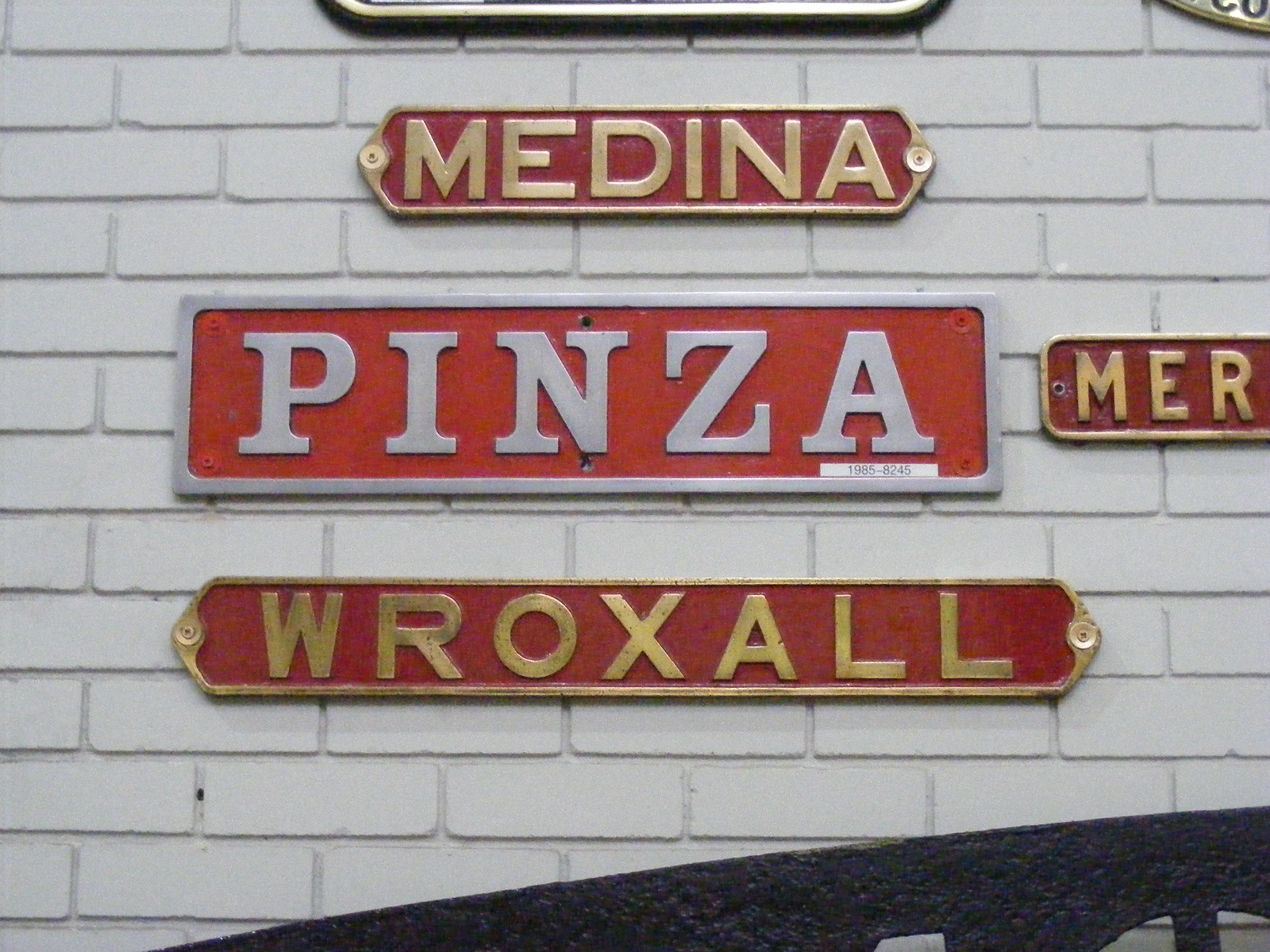This image depicts a white-painted brick wall adorned with several metal street signs. Prominently featured at the top is a red plaque with gold lettering that spells "Medina." Below it, there's another red sign, rimmed and lettered in silver, reading "Pinza." Further down, a longer and darker red sign with gold trim and letters spells "Roxul" (though one account misspells it as "Wroxall"). An additional partially visible sign to the right of "Pinza" reads "MER" and extends out of the frame. The lower right corner of the photograph hints at a potential entryway or possibly a bench, but the details are unclear. The posted signs evoke a decorative or directional purpose, unified by their vibrant red backgrounds and metallic accents.